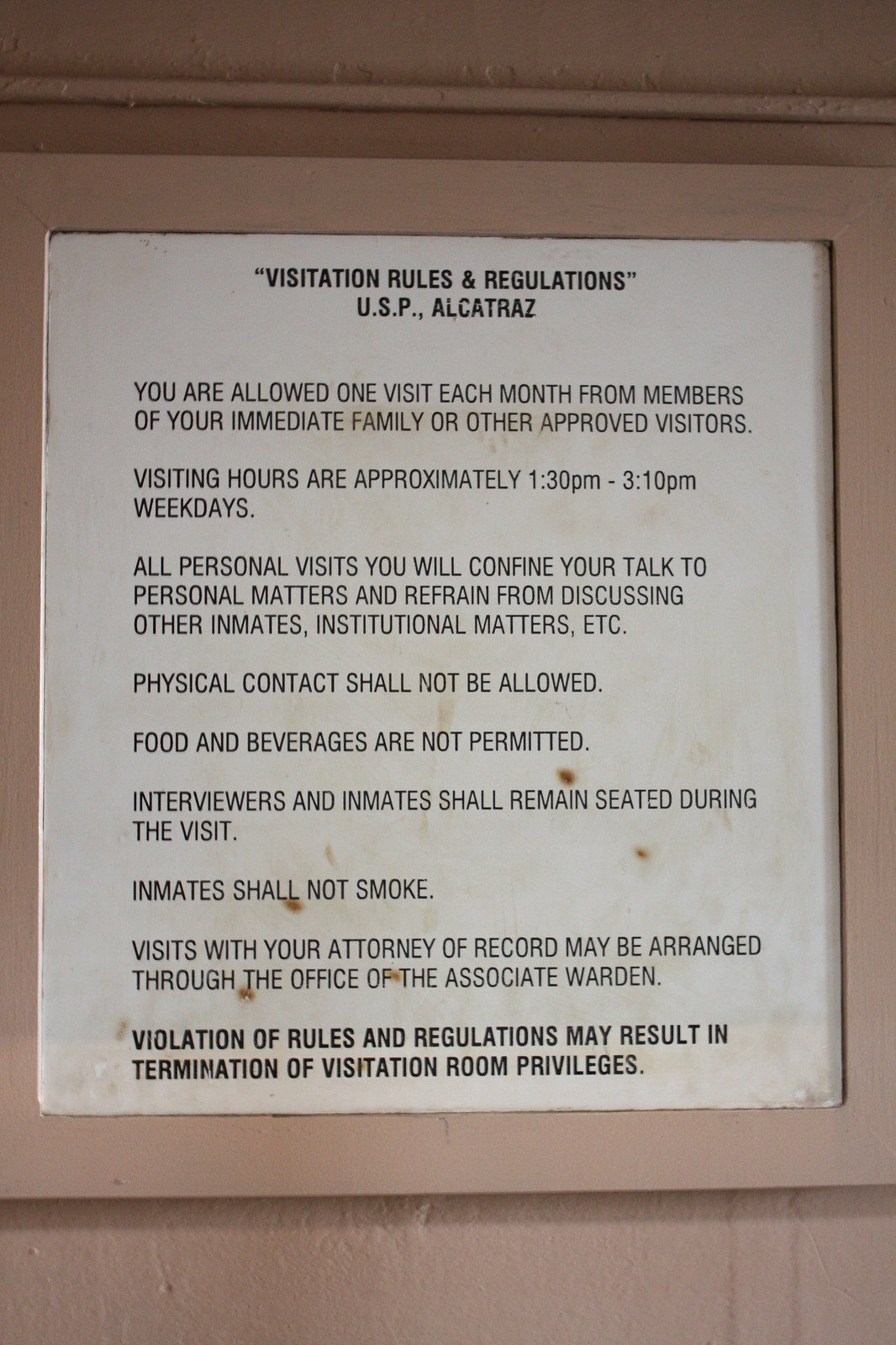The image features a framed list of rules, likely posted at the entrance to Alcatraz, set against a tan or beige background. At the top of the sign in quotes, in bold black capital letters, are the words "VISITATION RULES AND REGULATIONS." Below this, it states "USP. Alcatraz." The main body of the text reads:

- You are allowed one visit each month from members of your immediate family or other approved visitors.
- Visiting hours are approximately 1:30 p.m. to 3:10 p.m. on weekdays.
- During all personal visits, you must confine your talk to personal matters and refrain from discussing other inmates, institutional matters, etc.
- Physical contact shall not be allowed.
- Food and beverages are not permitted.
- Interviewers and inmates shall remain seated during the visit.
- Inmates shall not smoke.
- Visits with your attorney of record may be arranged through the office of the Associate Warden.

In bold black text at the bottom, it warns, "Violation of rules and regulations may result in the termination of visitation room privileges."